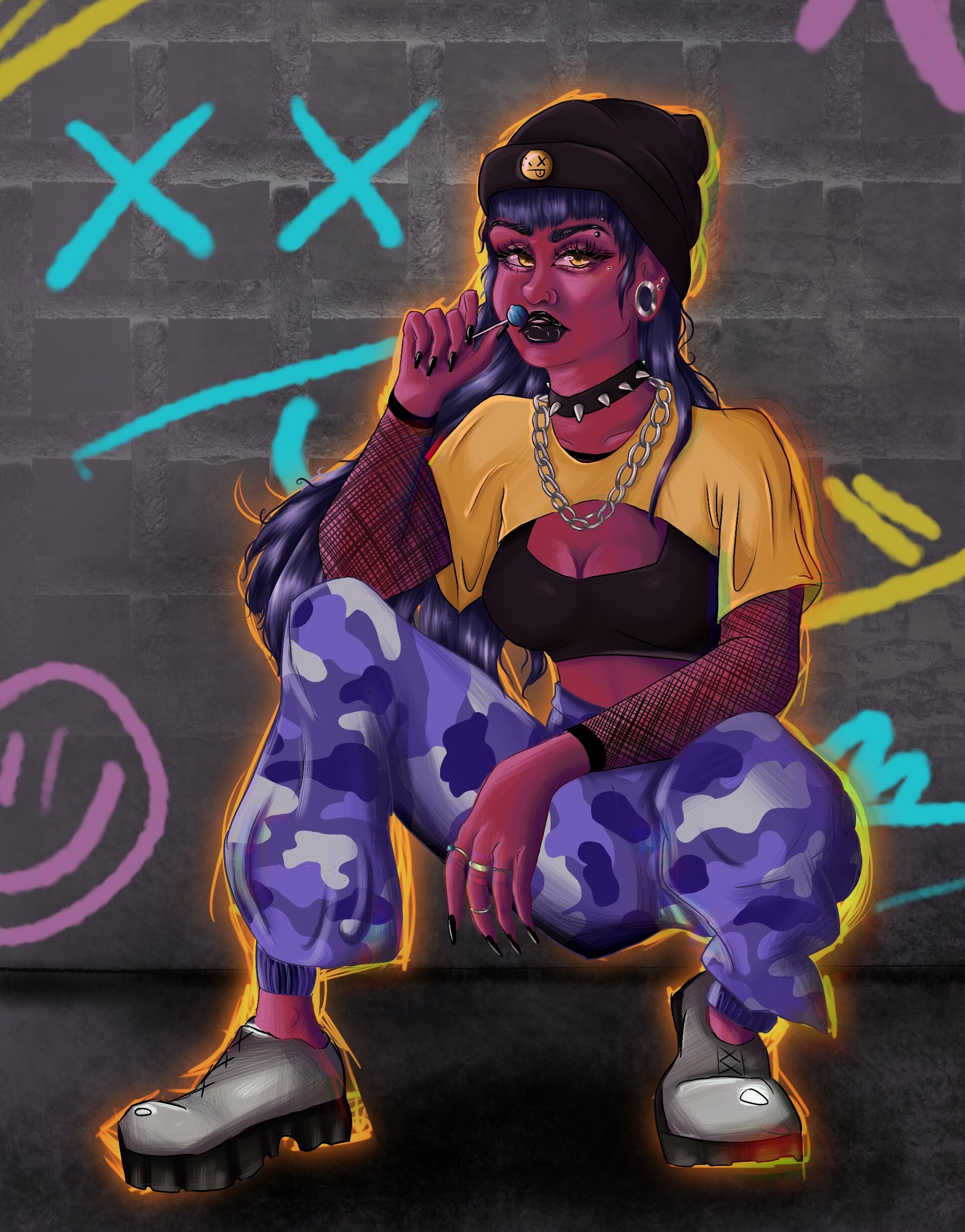In this vertical, cartoonish painting that appears AI-generated or animated, a woman is depicted squatting on the street, amidst vibrant street art. She wears striking purple camouflage-style pants with light and dark purple patterns, a yellow half-shirt partially revealing a black sports bra, and white shoes without socks. Her elaborate accessories include two necklaces, earrings, and an adornment in her swept-back dark hair. The woman’s makeup includes black lipstick, and she holds a blue lollipop up to her mouth with her right hand. She is positioned on a tic-tac-toe-like street painting with a prominent purple smiley face at the bottom left. Behind her, a brick wall serves as the backdrop, adorned with graffiti, including two light blue X's, yellow, turquoise, and pink markings scattered about, creating a rich, urban tapestry.